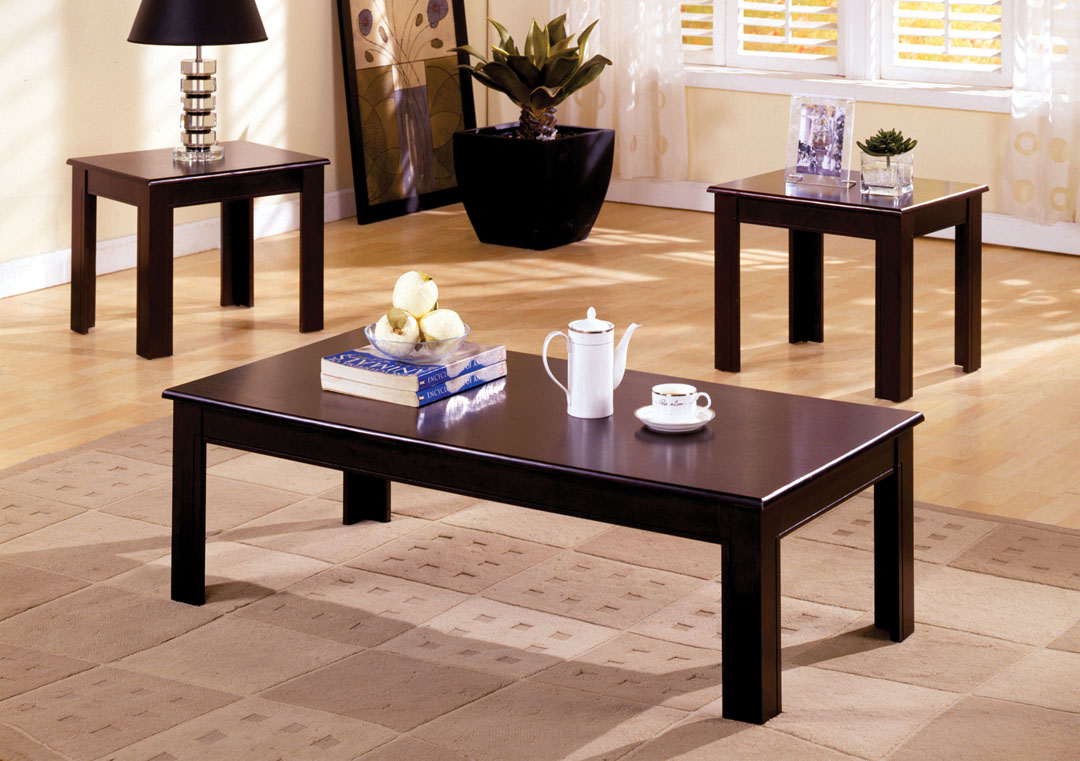The photograph features a meticulously staged, minimalist living room setup, likely intended for a catalogue or stock image. Central to the scene is a dark brown, highly polished coffee table set at a slight diagonal, adorned with a white porcelain teacup, saucer, and coffee pouring jug, and two blue books with some decorative items on top. Beneath the coffee table, there is a beige checkered area rug with a mix of lighter and darker brown patches, contrasting with the surrounding light wooden plank flooring.

To the left in the background stands a smaller end table topped with a crystal lamp and a black lampshade, the lamp being slightly cut off by the top edge of the image. On the right, another matching end table displays a glass photo frame and a small square glass container with a dark green short plant. The back left corner hosts a black flowerpot with a small palm-like plant, its dark green leaves pointing upward at a 45-degree angle. Behind the plant, a piece of abstract artwork leans against the yellow wall, which also features a window with California shutters, letting in daylight and giving the scene a warm, inviting glow.